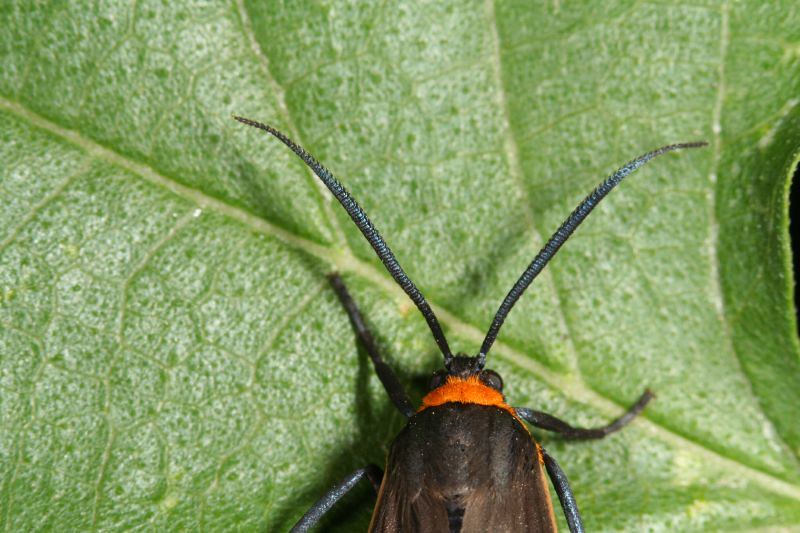The image showcases a highly detailed, close-up shot of an insect perched on a large green leaf. The vibrant leaf, which occupies the majority of the frame, displays intricate details such as veins and speckles, transitioning from light to dark green. The insect, likely a moth, is only partially captured but is richly detailed. It features bright orange, fuzzy fur on its head, two large black antennae, and black legs. Its furry face has prominent black eyes, and you can also see the start of its thick brown wings just behind the head. The insect appears to be resting on the leaf, potentially crawling or feeding. The lighting and sharp focus suggest professional photography, emphasizing the insect's and leaf's textures. The predominant colors in the image include shades of green, brown, black, orange, and white.